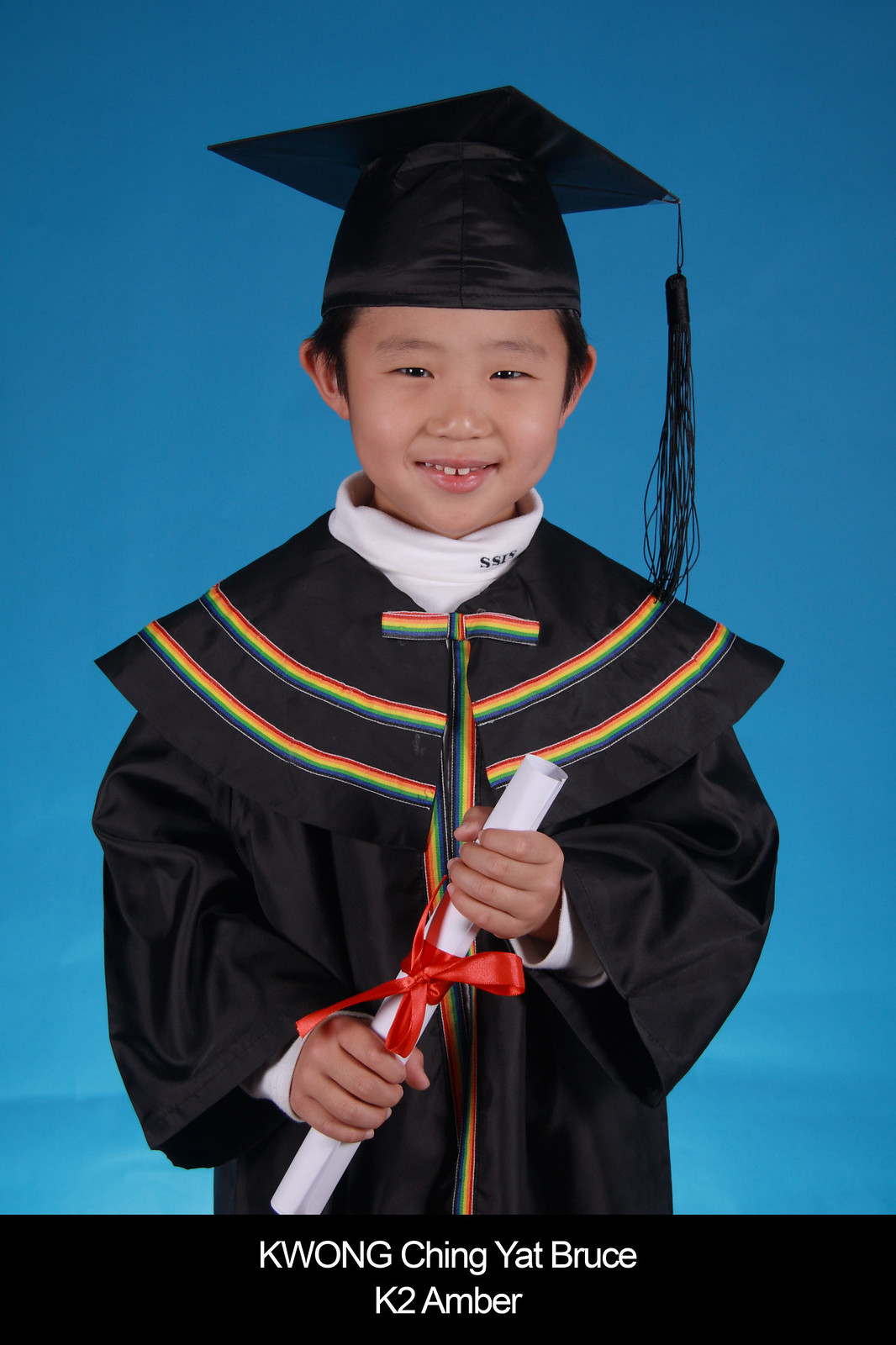This is a detailed portrait of a young, smiling boy celebrating his graduation, likely from kindergarten or elementary school. He stands in front of a blue background that transitions from a darker shade at the top to a lighter hue at the bottom. The blue backdrop highlights a horizontal black bar at the base of the image, which displays the text "Kwong Ching Yat Bruce" in white letters, followed by "K2 Amber." The boy is wearing a traditional black graduation cap with a black tassel on the right side, paired with a matching black gown adorned with small rainbow stripes across the shoulders and down the center. In his hands, he proudly holds a rolled white diploma tied with a red ribbon, gazing directly at the camera with a joyful expression. The young graduate appears to be Asian, adding to the warmth and excitement of this milestone moment captured in the photograph.